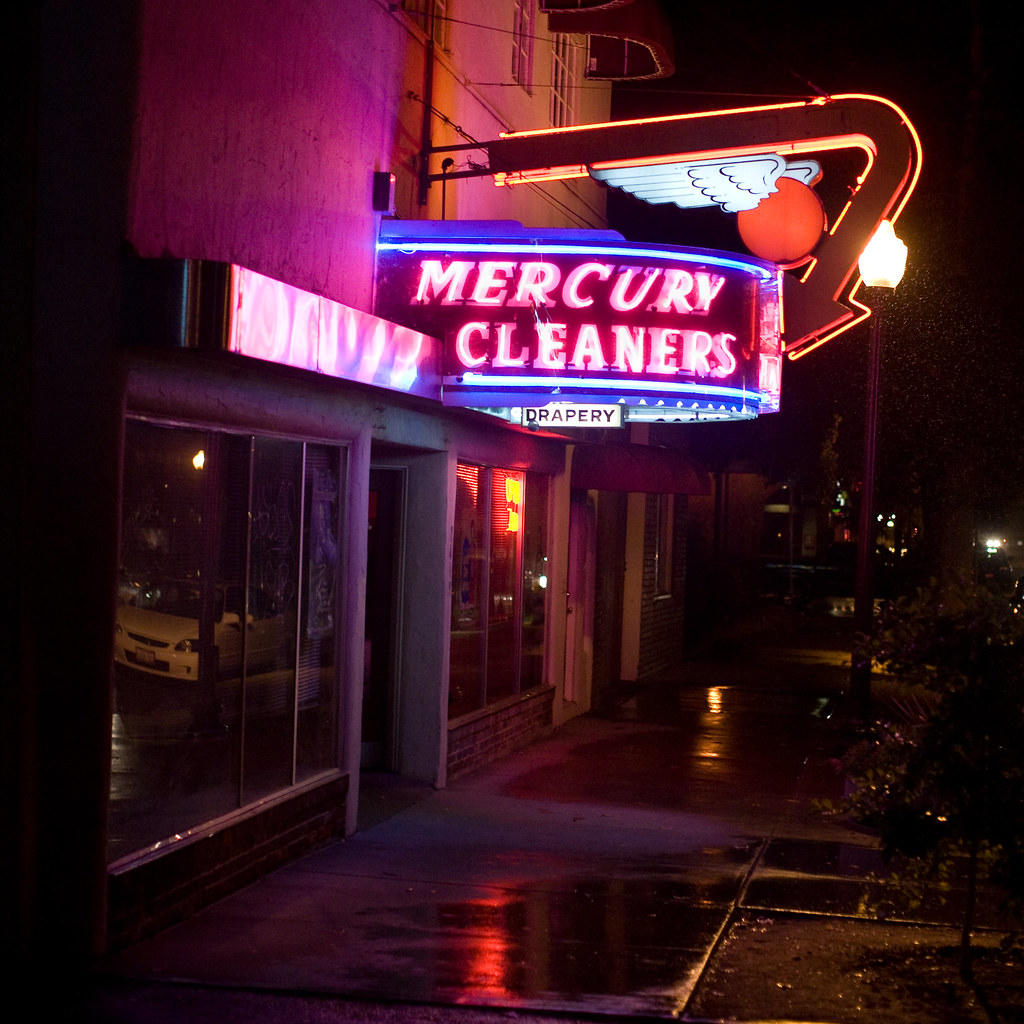The image captures a neon-lit storefront at nighttime, facing the street. The business, identified by a neon sign that reads "Mercury Cleaners" in pink, is framed by a reflective, glass-filled building facade. The glass reflects the wet sidewalk and the street, which features parked cars, including a visible white car. The neon sign is topped with a vivid blue line and an illuminated arrow that curves downwards and points directly at the "Mercury Cleaners" sign. This arrow is inset with a red circle accompanied by two white wings, adding a distinctive visual element. Below the main sign, a small white sign reads "Drapery" in black lettering. To the right of the entrance, a tree and a shrub are present, possibly within a dirt bed, further indicating a recent rainfall evidenced by the glistening, wet sidewalk.